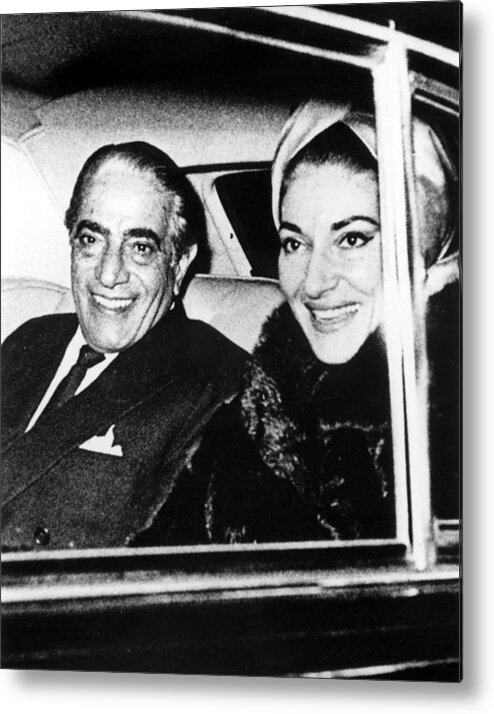A classic black and white photograph, possibly dating back to the mid-1960s to 1970s, captures a joyful moment inside the backseat of a vintage car. The image, taken through a partially lowered window, reveals the silver edges and trim of the dark-colored vehicle. In the foreground, a woman sits to the right, donning a light-colored headscarf that reveals her dark, pulled-back hair, and a luxurious black fur coat that envelops her neck. Her pronounced chin and bright smile emphasize her cheerful demeanor. Beside her, an older man, dressed impeccably in a dark suit, white shirt, dark tie, and a flamboyantly folded pocket square, gazes directly at the camera with a broad smile. The soft leather seat they are seated on accentuates the car's elegant interior, while the dark, blank view through the rear window adds a mysterious touch. The photograph exudes a sense of glamour and happiness, hinting at the couple's possible fame and the notion of this being a candid, possibly paparazzi, shot from an era gone by.